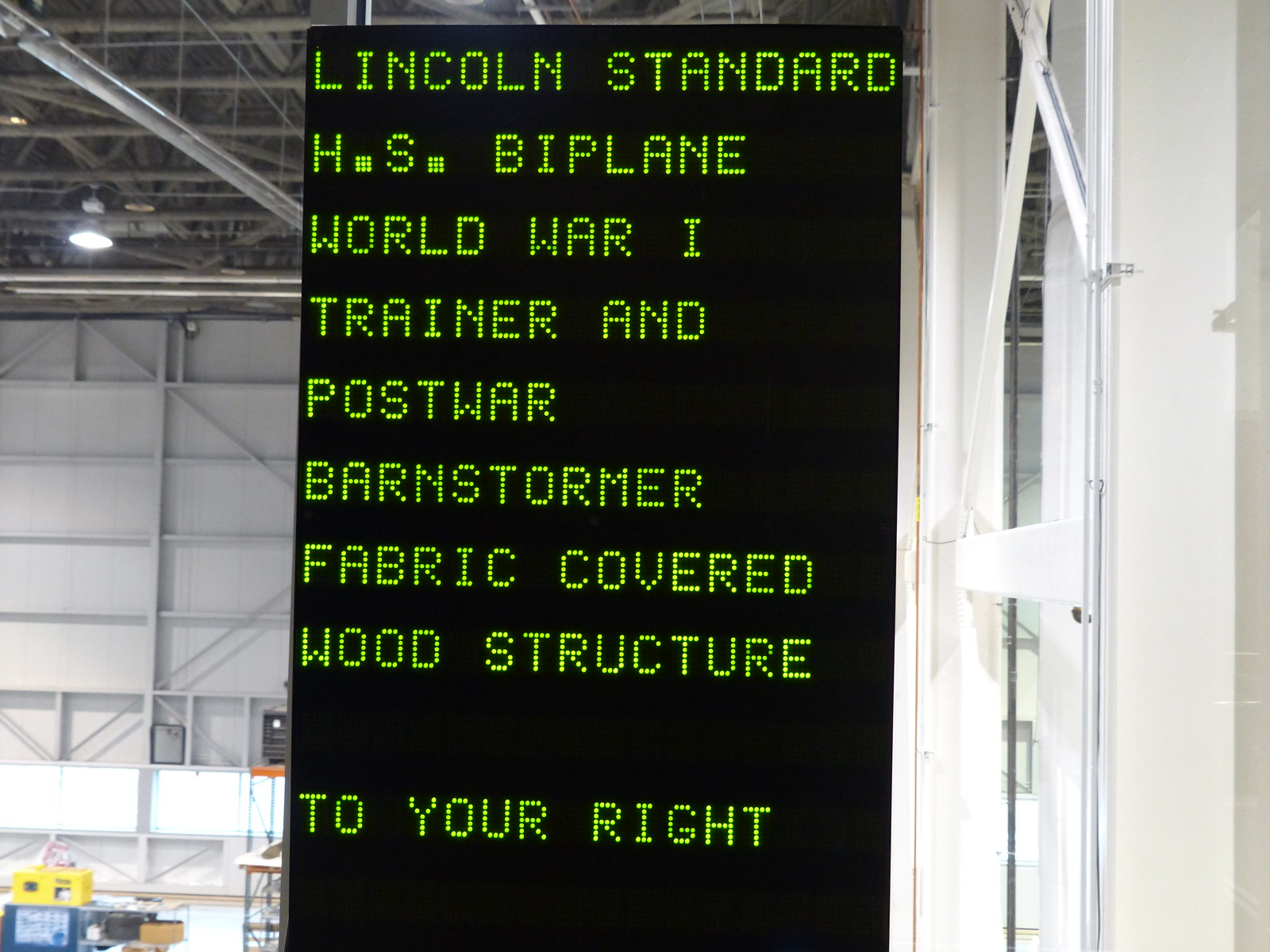The image depicts the interior of a large warehouse-like building, potentially a museum, with high ceilings supported by metallic beams and ample lighting. A prominent black electronic sign juts out from the wall, displaying detailed green-text information in a digital font reminiscent of Family Feud's style. The sign reads: "Lincoln Standard HS biplane, World War One trainer and post-war barnstormer fabric-covered wood structure to your right." The space below shows yellow and blue objects, possibly construction vehicles and scaffolding, though there are no visible people or actual airplanes in sight. The white walls and matching metal structures contribute to the spacious, industrial feel of the building.